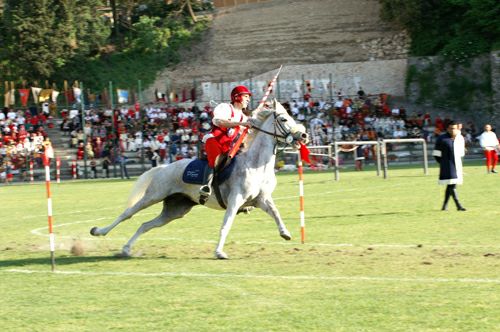The image captures an outdoor equestrian event featuring a white horse in mid-gallop with dirt and grass being kicked up beneath its hooves. The horse, adorned with a dark brown harness and a blue saddle blanket, carries a rider dressed in a distinctive red and white uniform with red pants, a white shirt, and a red helmet. The rider, who appears to be a jockey or a jouster, is holding a red and white spear-like object and leaning sideways as the horse runs. On the course, the horse is navigating between two red and white poles, adding to the sense of action and competition. In the background, an assortment of spectators can be seen seated in outdoor grandstands, with some standing on the field, including a judge in a black and white uniform. Among the crowd, various multi-colored flags are waving, and behind them stretches a landscape of green grass and a dirt hill dotted with trees. The scene is brightly illuminated by daylight, capturing the dynamic and somewhat chaotic intensity of the moment, with the horse's stance indicating a lack of poise as it maneuvers through the course.